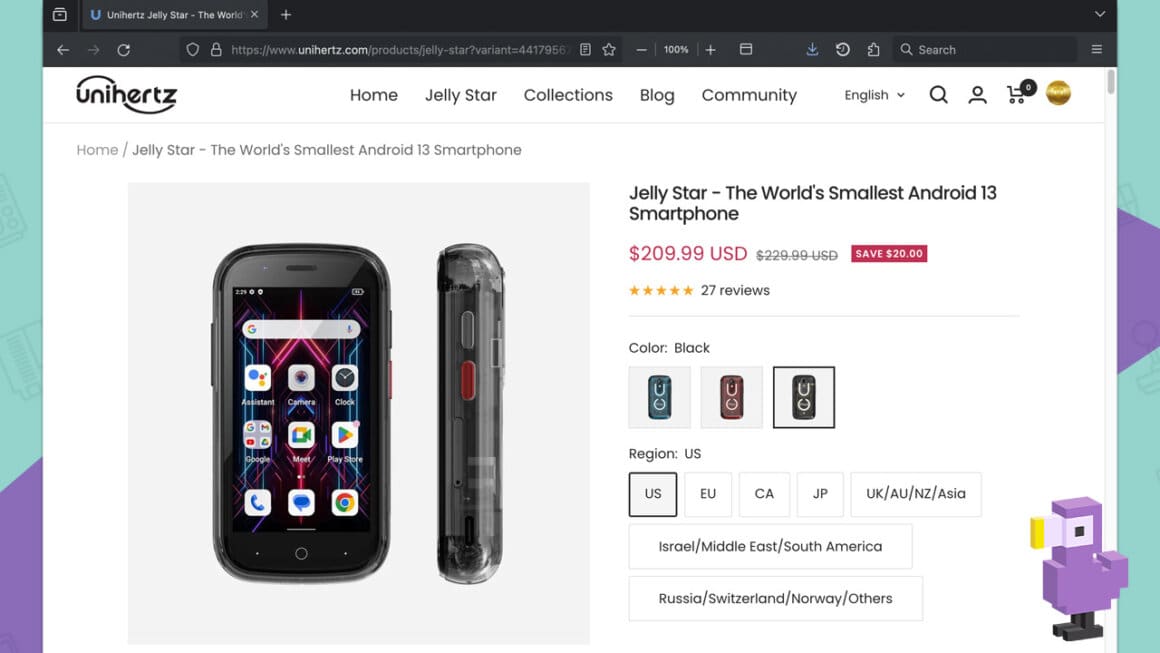This screenshot showcases a web browser with a single tab open, indicated by a visible padlock icon in the top left corner, signifying a secure connection. The tab is labeled "unihertzjellystar-the-world." Below the tab bar, standard navigation elements are visible, including left and right arrows for navigation, a refresh circle, and several icons. The URL displayed is "https://www.unihertz.com/products/...", with the domain highlighting the official Unihertz website.

The toolbar features icons for bookmarks, screen size adjustment set at 100%, a download button, a back-in-time option, extensions, a search bar, and the main menu. The webpage itself has a white background and prominently displays the Unihertz logo in the top-left corner, accompanied by a navigation menu that includes links for Home, JellyStar, Collections, Blog, Community, language selection (English), a search icon, an account icon, a shopping cart icon, and a distinct yellow circle icon.

Central to the page is a feature banner highlighting the text "JellyStar – The World's Smallest Android 13 Smartphone," accompanied by a brief description. This section emphasizes the JellyStar's unique selling points and seeks to engage viewers with the product's key features.